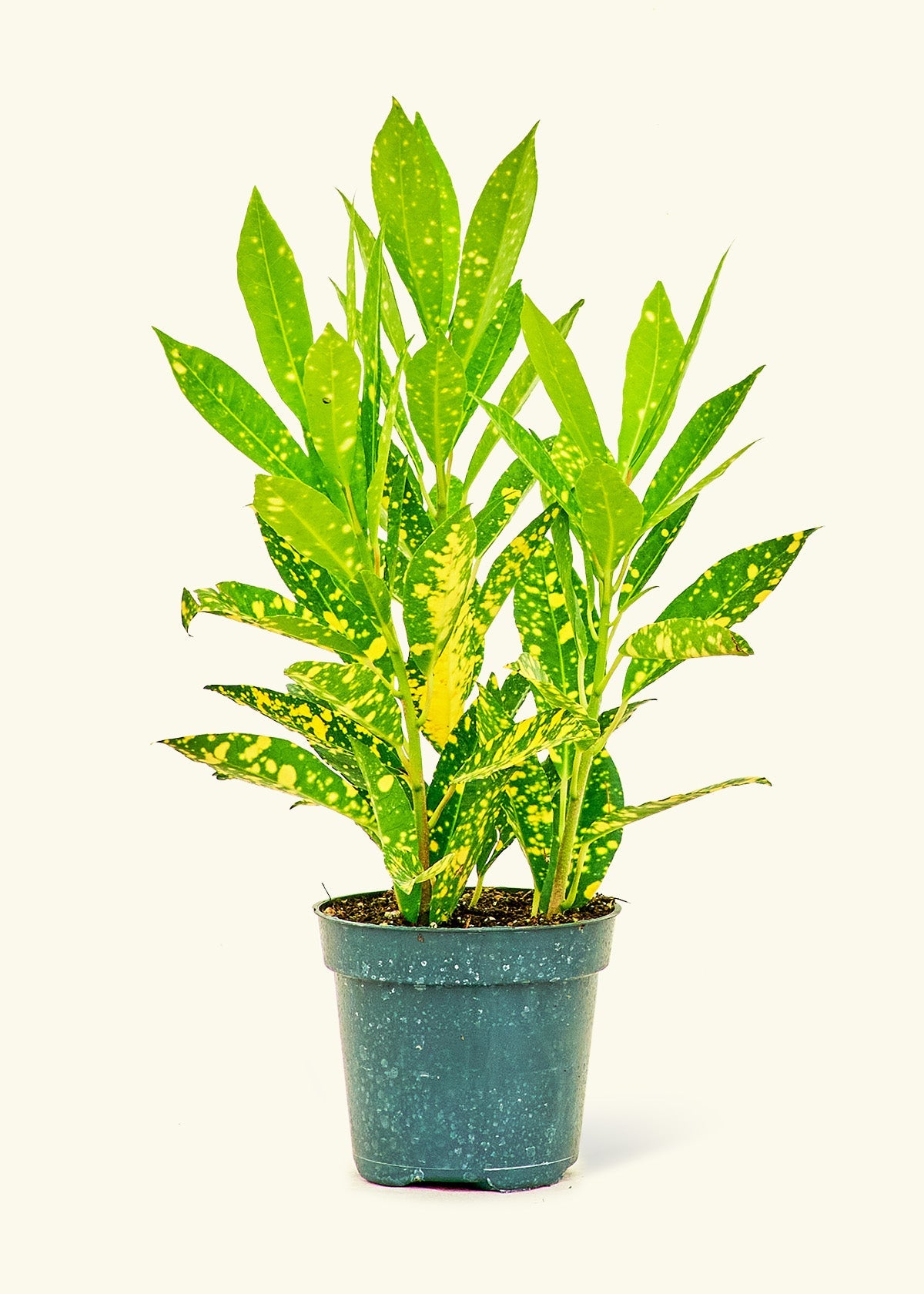This image depicts a vibrant potted plant positioned front and center against a seamless light tan or white background, creating an indistinct separation between the floor and the wall. The plant, which rises approximately two to three feet from its base, showcases long green leaves adorned with yellow speckling, more concentrated towards the bottom. The plant sits in brown soil within a traditional, blue or dark green plastic pot that features some flecks of white and slight dirt and grime, emphasizing its well-used nature. The healthy appearance of the plant, coupled with its detailed speckled leaves and simplistic, indistinct background, clearly spotlights the plant as the focal point of the image, suggesting its potential use in a context related to plant care or identification.